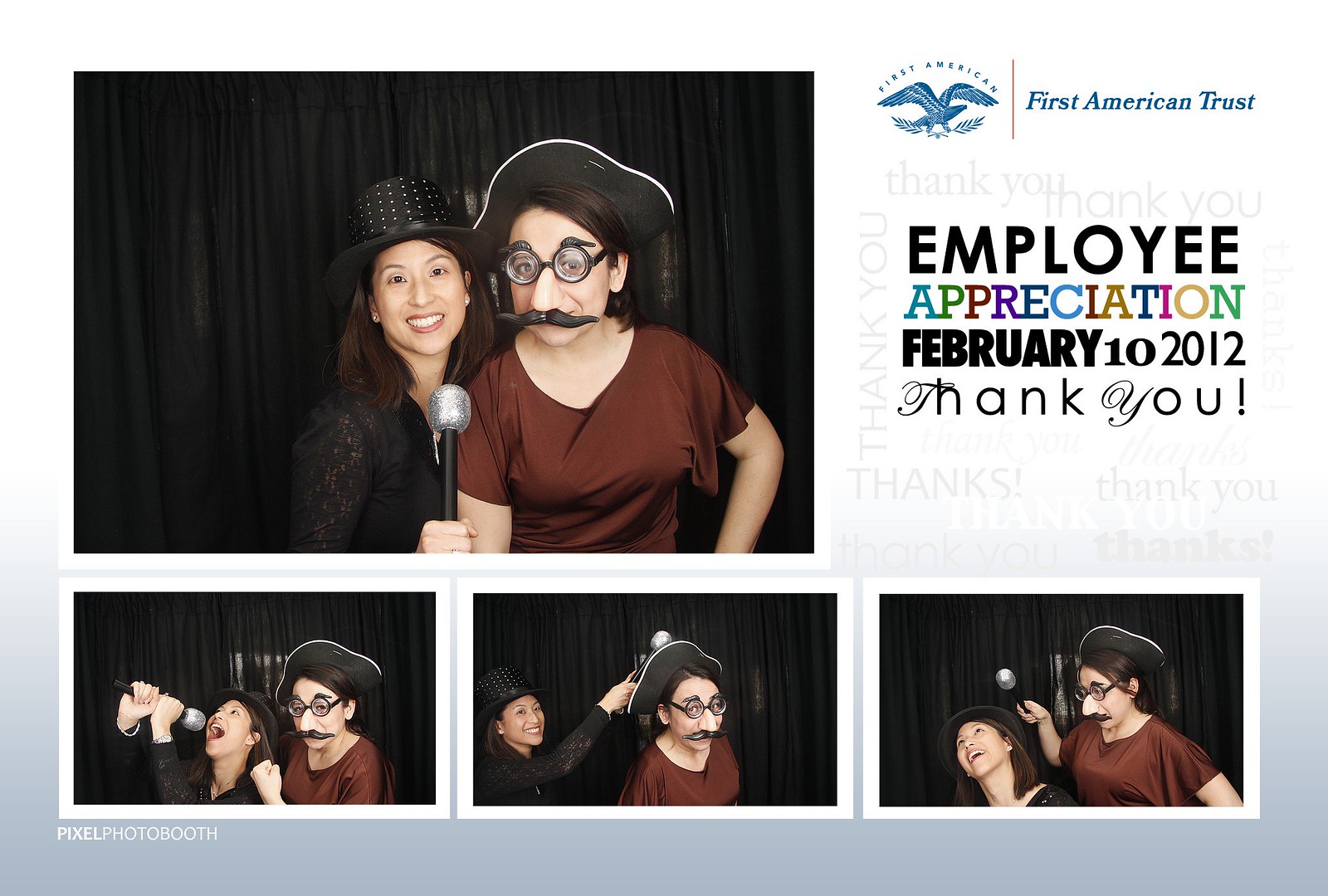This image, likely taken from a website, showcases a collage centered around an event held by First American Trust. At the top, the logo of First American featuring a falcon is prominent, followed by a red vertical line and the text "First American Trust." Below this, the heading "Employee Appreciation" stands out with colorful lettering, followed by the date "February 10, 2012," and a repeated "thank you" message in the background on the right-hand side.

The central image displays two women dressed in playful attire, seemingly celebrating a themed event, possibly Halloween. The woman on the left sports a black hat with white spots, long brown hair, and a black top, while holding a glittery or fake microphone. The woman on the right is wearing a black pirate hat, oversized googly glasses, a fake nose, a mustache, and a maroon-colored top.

Beneath the main picture are three smaller photos showing the women in various humorous poses: in the first, the woman on the left appears to be singing into the microphone while the other poses with a mock punch; in the second, the woman on the right interacts with the hat of the first; and in the third, the two continue their playful antics. The collage captures the spirit of camaraderie and fun at the employee appreciation event.